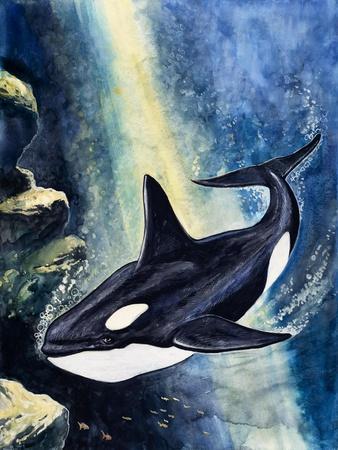The vertical image depicts an underwater ocean scene featuring an orca, also known as a killer whale, swimming deep beneath the surface. The orca's classic black and white color pattern is evident, with its predominantly black body contrasted by a white underbelly and a distinct white oval spot above its left eye, which could be mistaken for its actual eye. The whale is portrayed in a side view, seemingly moving downward in a yellow sunbeam that illuminates its sleek body. Surrounding the orca are numerous air bubbles, notably around its mouth and fins, enhancing the sense of movement. To the left of the whale is a rock outcropping, and beneath it, tiny, indistinct fish swim through the bluish water. The artwork, executed in an impressionistic style with either colored pencils or watercolors, captures the serene and majestic nature of the underwater world with gentle hues and a focus on the graceful form of the orca.